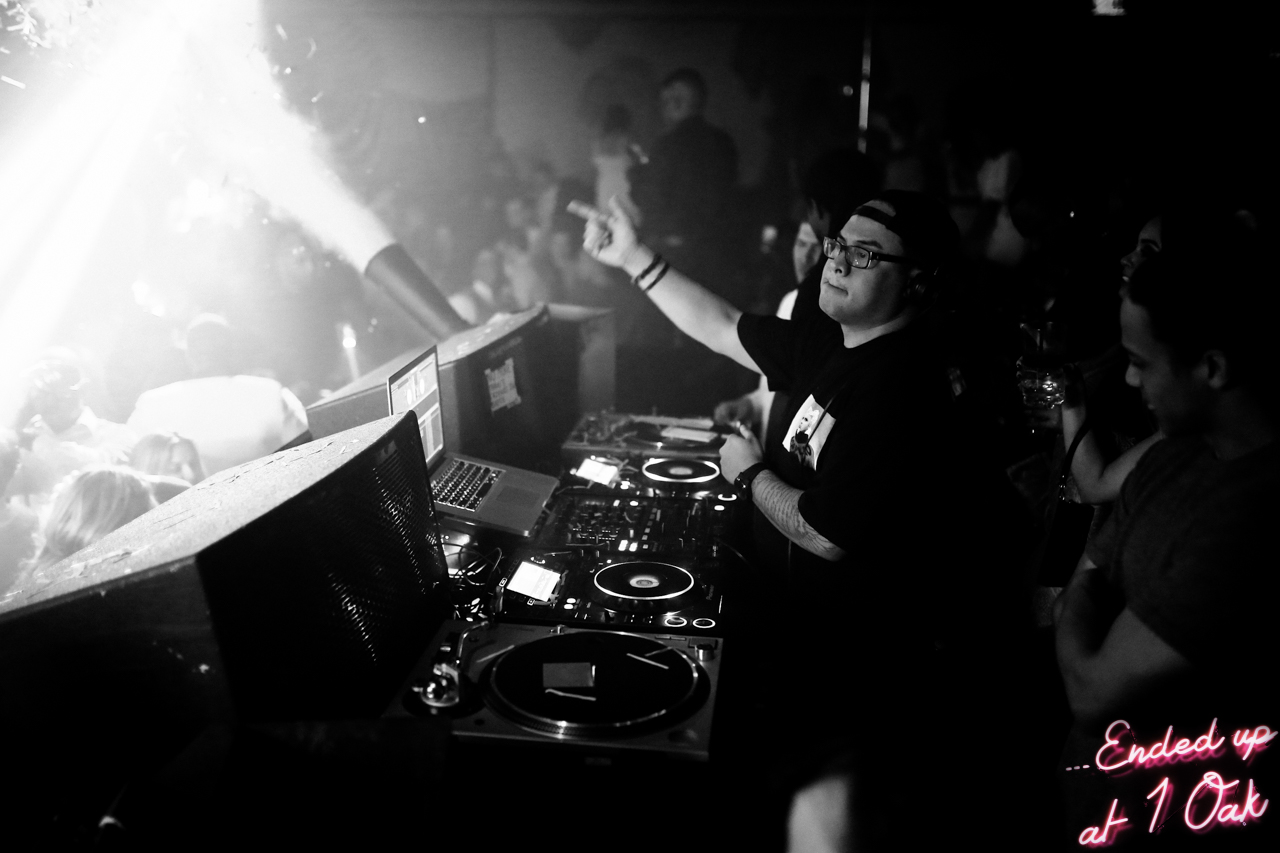In this black and white photograph, a lively party scene unfolds at the renowned nightclub One Oak, identifiable by the pink-outlined, cursive text "…ended up at One Oak" in the bottom right corner. The energetic atmosphere captures a DJ at the helm, standing in front of turntables and a silver laptop. With both hands raised in the air, he's engulfed in pyrotechnics and smoke effects, heightening the festive ambiance. The DJ, sporting a backwards cap, black shirt with an indistinguishable logo on the left breast pocket, black-framed glasses, two wristbands on his right hand, and a watch on his left, is surrounded by an enthusiastic crowd, though the dark setting makes their details hard to discern. The equipment before him is black with silver buttons, adding to the sleek, lively aesthetic of the scene. The walls appear white, contributing to the stark contrast and energetic vibe of this memorable night at One Oak.